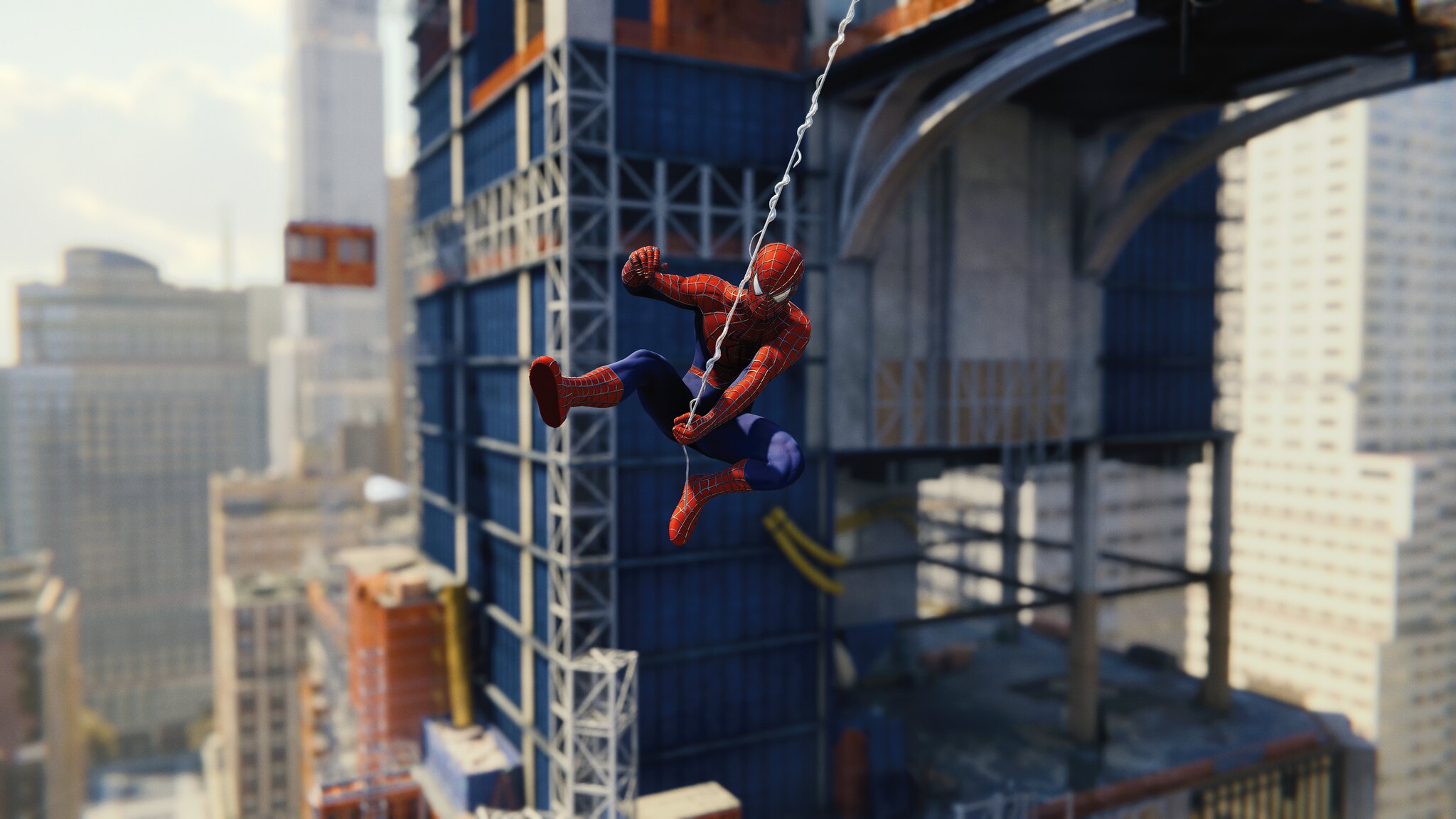In this striking image, likely from a video game or animated movie, Spider-Man is suspended mid-air in his iconic red and blue costume. The dynamic scene captures him swinging from a single strand of spider web that dangles from a bridge overhead, with the web prominently running over his right shoulder and held tightly in his left hand. His right arm extends outward, suggesting his readiness to propel himself forward. Spider-Man's distinctive white eyes stare directly at the camera, adding intensity to the moment. The background showcases a detailed cityscape, featuring a large blue skyscraper under construction with a balcony extending outward, and additional tall buildings on either side, including some grayish white skyscrapers. The partially visible sky, tinged grayish-white, reinforces the sense of height and vastness in the image.